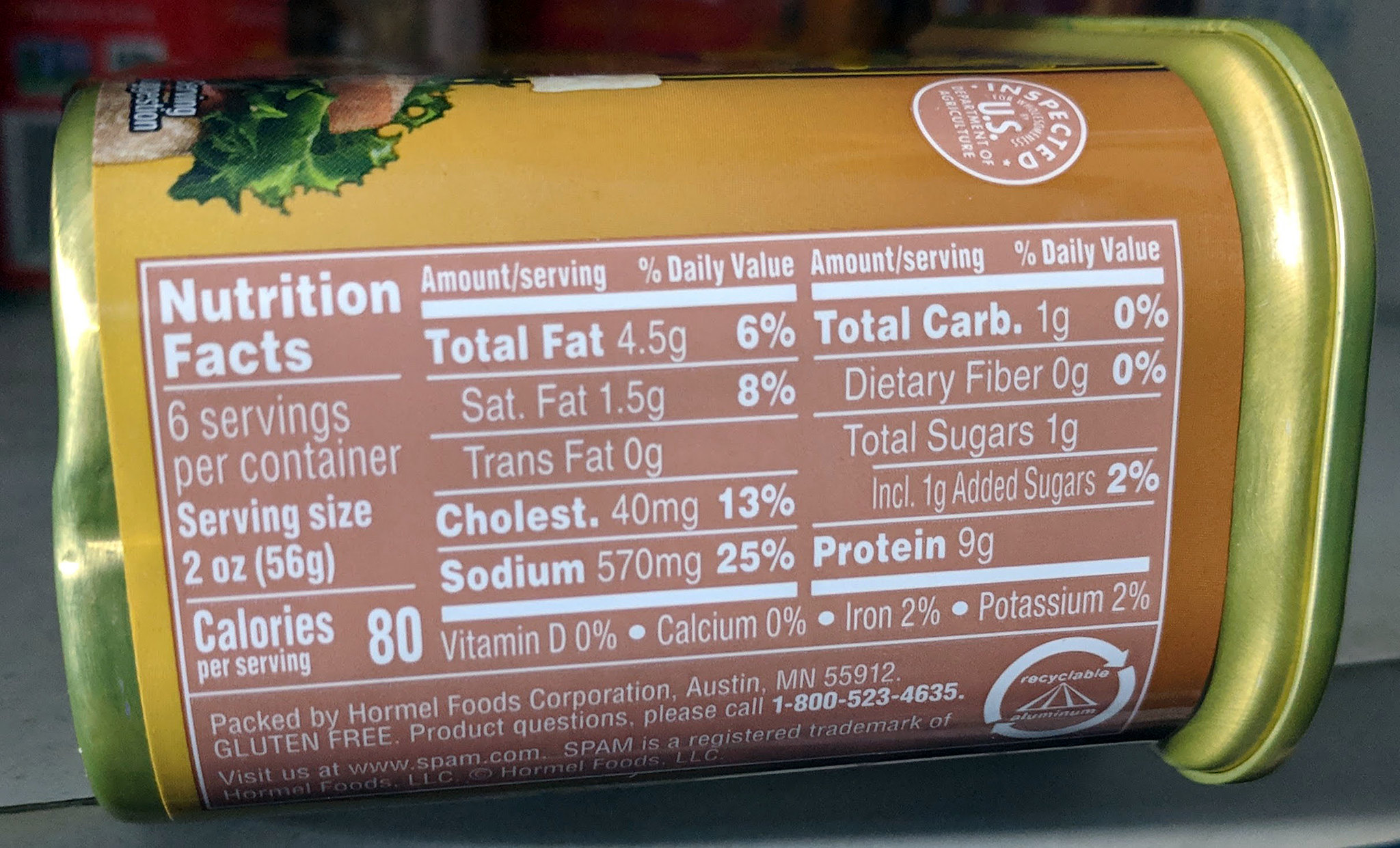This detailed close-up photograph features a rectangular metal can of Spam with a golden top and bottom. The can prominently displays a bright, salmon-colored label adorned with white text. On the left side of the label is an image of the Spam product itself, depicted as a brown, ham-like piece with darker brown or red sides, accompanied by dark green leaves with lighter accents for garnish.

Central to the image is the nutritional information label, which begins with “Nutrition Facts” in white text. Highlighted details include: six servings per container, each serving size being two ounces (56 grams), providing 80 calories per serving. The total fat content is 4.5 grams (6% of daily value), with 1.5 grams saturated fat (8% of daily value), and 0 grams trans fat. The cholesterol content is stated as 40 milligrams (13% of daily value), and the sodium content as 570 milligrams (25% of daily value). Carbohydrates total 1 gram (0% daily value), dietary fiber 0 grams, total sugars 1 gram (including 1 gram of added sugars, equating to 2% daily value), and protein 9 grams. Additional nutritional details reveal that the product contains 0% Vitamin D, 0% Calcium, 2% Iron, and 2% Potassium.

The label also indicates that the product is inspected by the U.S. Inspection Service and is packaged by Hormel Foods Corporation in Austin, Minnesota, with a contact number for product inquiries provided at the bottom.